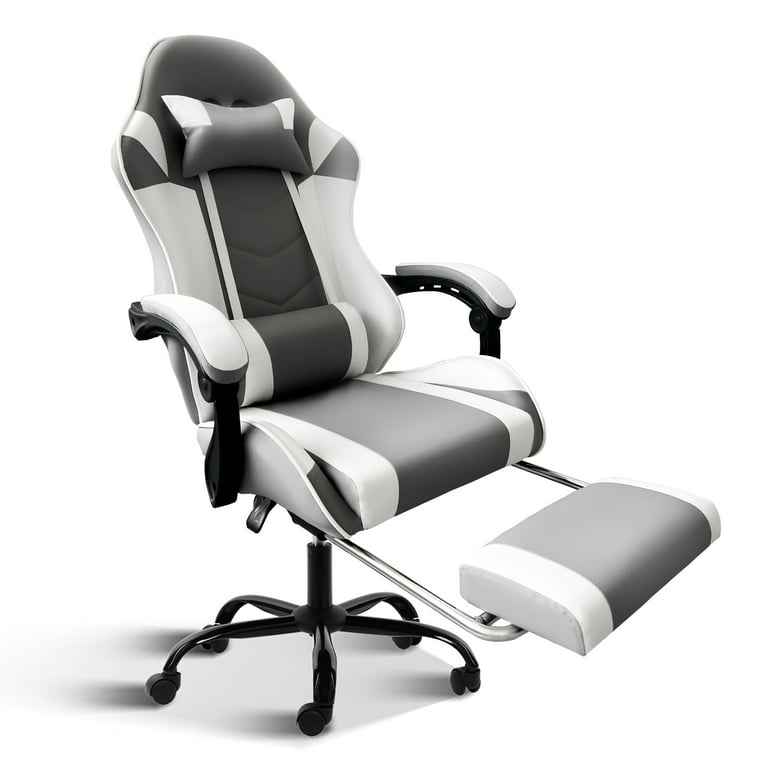The image showcases a high-quality gaming or office chair with a modern, racer-style design. The chair features a tall, contoured back with a distinctive wave pattern, culminating in a rounded top, and comes with both a headrest pillow and a lumbar support pillow. It has padded armrests and an adjustable footrest on an extender bar, enhancing comfort for extended use. The chair boasts a sophisticated color scheme with a dark gray stripe running down the middle and white flanking the exterior sides. The seat features standard cushions with additional thigh-support cushions, primarily in white with black accents on the lower part. The chair's base includes five solid rubber rollers attached to black metallic legs, ensuring stability and mobility. Adjustable controls on the right side allow for seat height modification. This product image, either a digital rendering or a high-resolution photograph, is presented on a white background with a subtle drop shadow, suggesting a polished and potentially high-end chair.